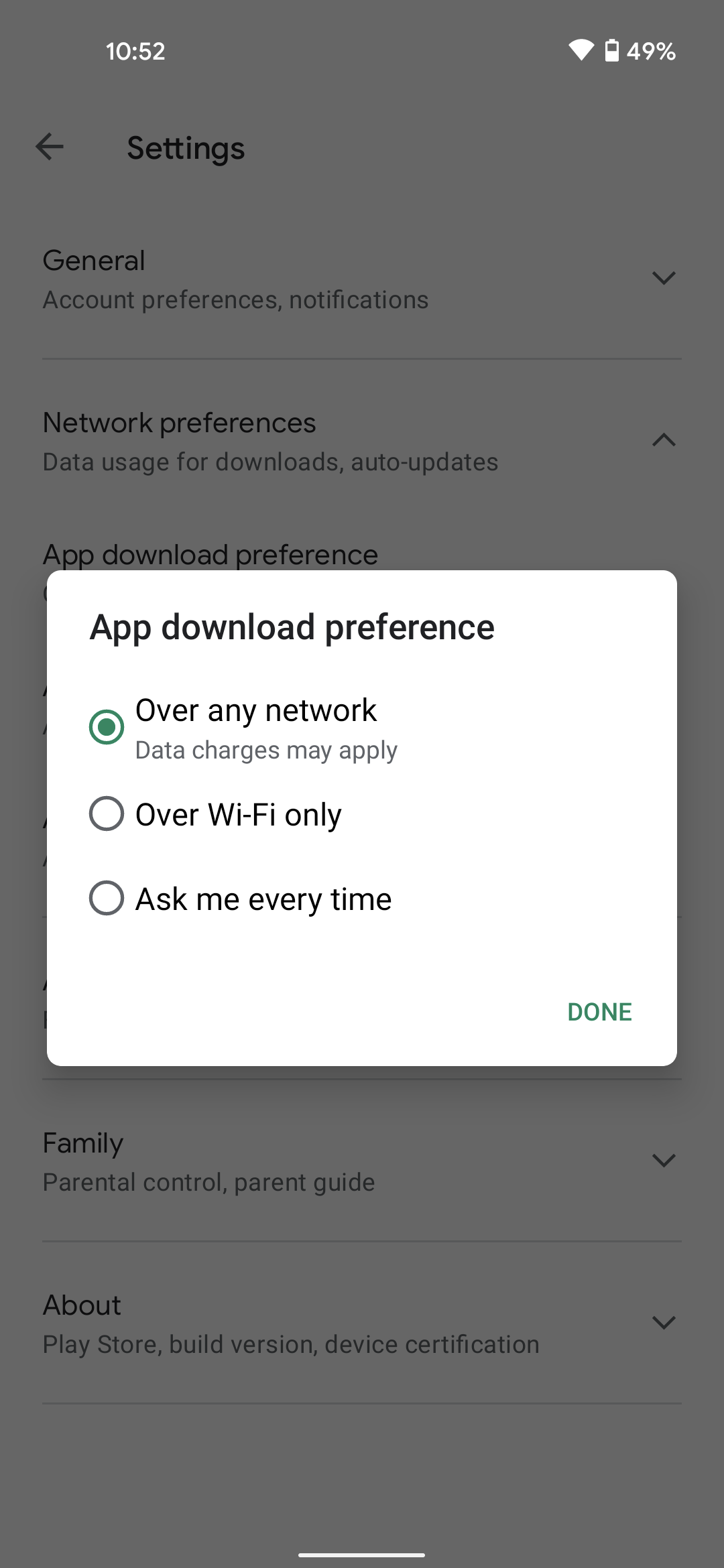This screenshot, captured on a mobile phone, shows the device's settings page partially obstructed by a pop-up menu. The timestamp displayed at the top reads 10:52. In the upper right corner, icons indicate no mobile signal, full Wi-Fi connectivity, and a battery level at 49%. The background settings screen, greyed out due to the pop-up, features a back arrow labeled "Settings" at the top. Visible options include "General," "Network Preferences," and "App Download Preferences," while other options are obscured by the pop-up. Towards the bottom, partially visible options include "Family" and "About."

The pop-up menu presents three choices for app download preferences: "Over any network (data charges may apply)," "Over Wi-Fi only," and "Ask me every time." At the bottom of the pop-up is a "Done" button, allowing the user to close the menu and return to the greyed-out settings screen behind it.